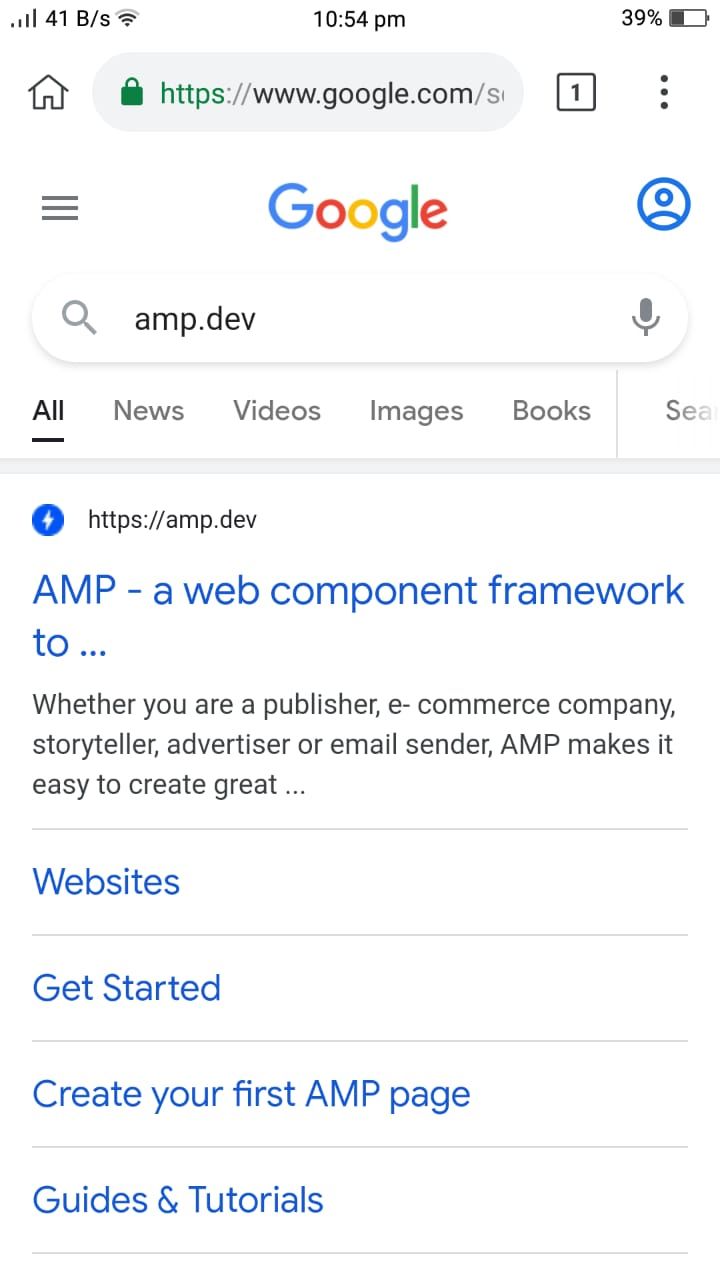A mobile phone displays a Google search result for "amp.dev" at 10:54 p.m., with a 41B/s data signal and a Wi-Fi logo in the upper left corner, and a 39% battery life indicator in the upper right corner. The white Google search bar at the top features a gray magnifying glass icon and a microphone icon for voice search. The search result highlights the AMP (Accelerated Mobile Pages) website, described as a web component framework beneficial for publishers, e-commerce companies, storytellers, advertisers, and email senders. Below the main description, blue link options for "Get Started," "Create Your First AMP Page," and "Guides and Tutorials" are separated by gray lines, making them easily distinguishable as clickable items.